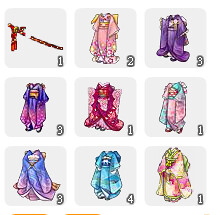The image consists of nine small, numbered illustrations arranged in a 3x3 grid, each set within a white square against a gray background. The illustrations primarily showcase different outfits resembling kimonos or yukatas, with rich, diverse colors. The numbering in the boxes follows a sequence: 1, 2, 3 in the first row; 3, 1, 1 in the second row; and 3, 4, 1 in the third row. 

In detail, the top-left illustration appears to contain a red sash or sword in its sheath. Moving right, the second and third images display a fluffy pink outfit and a purple dress with an additional wrap, respectively. Within the second row, the first illustration depicts an outfit with a purple top and blue bottom, followed by a design with red in the center and pink edges. The final illustration in this row is a blend of blue and pink hues.

In the third row, the first illustration shows an extensive wrap covering the entire figure, transitioning from blue at the top to purple at the bottom. The middle box contains an outfit in shades of greenish blue transitioning to lighter blue. The final illustration concludes with a light dark pink outfit.